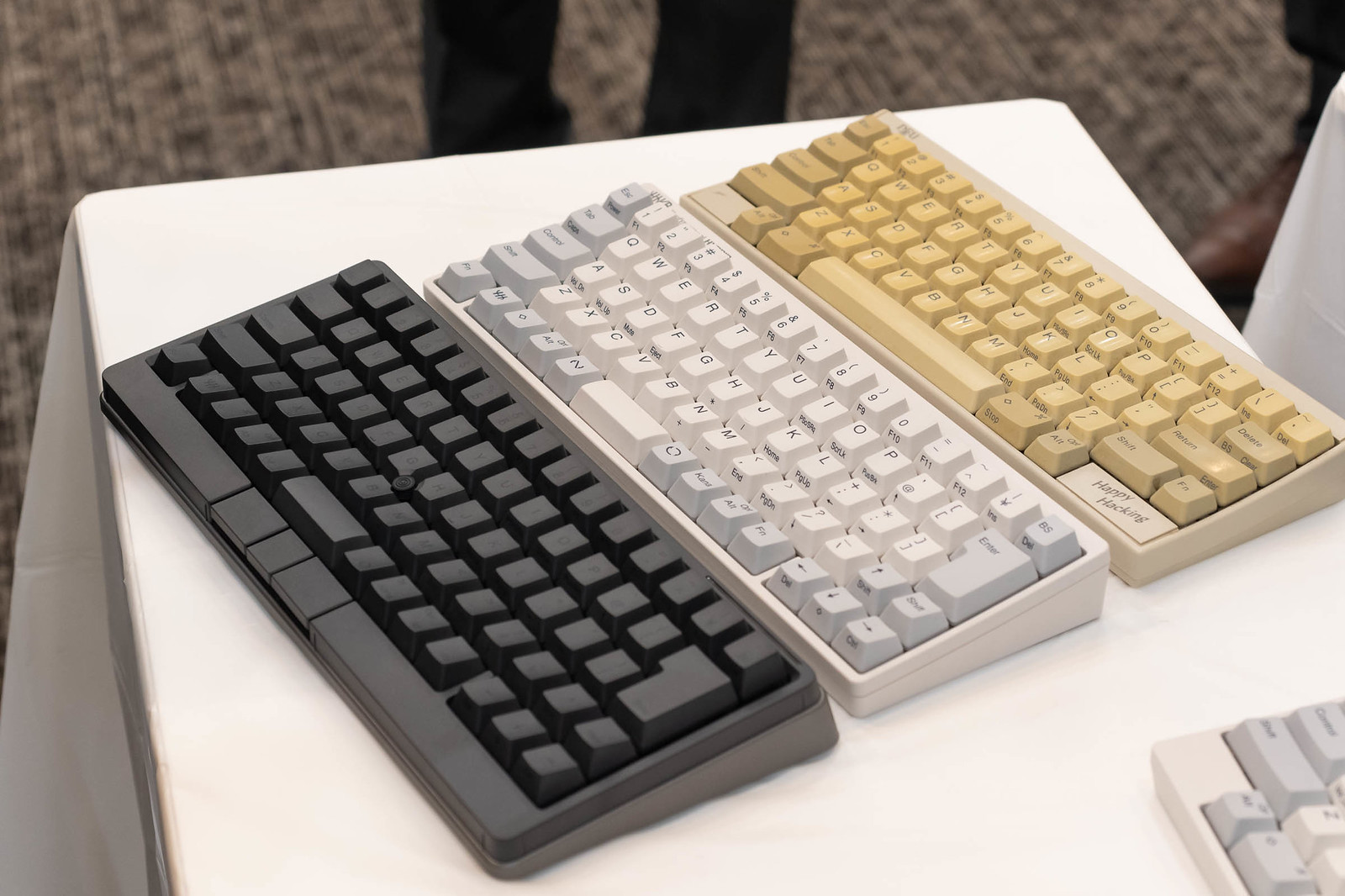This color photograph captures a scene featuring a white-topped desk, possibly draped in a cloth, with three different computer keyboards arranged diagonally from the bottom left to the upper right-hand corner. The bottom-most keyboard is entirely black, featuring no markings on its keys. The central keyboard is predominantly white with some keys, like Enter, Shift, and Backspace, highlighted in gray. The top-most keyboard is a yellowed, aged IBM model with a tan and ivory coloring. In the bottom right corner, part of another beige-colored keyboard intrudes into the frame. Just beyond the table's edge, two legs clad in dark pants suggest a person standing and observing the scene. The floor beneath features a patterned carpet with a commercial style, adorned in tan, cream, and brown tones, resembling an oriental rug. This image evokes a sense of a keyboard enthusiast's collection display.